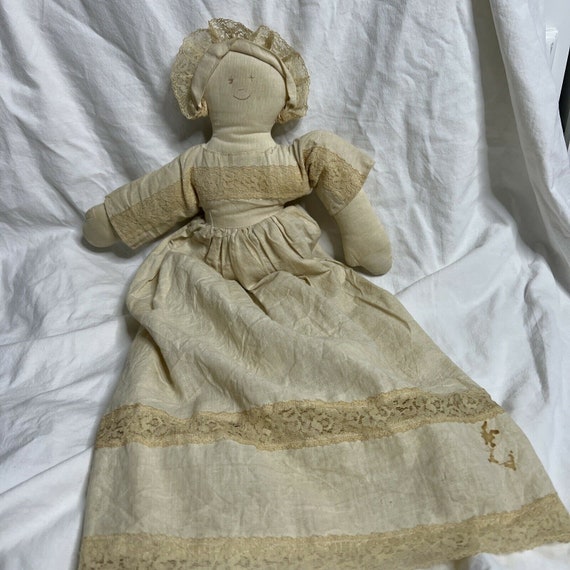This photograph features an antique, handmade fabric doll, possibly from the Victorian era, resting on a white sheet backdrop. The doll, appearing aged and discolored to a dingy yellow-tan color, is constructed from a stuffed cotton material. It is dressed in a voluminous, full skirt that includes two aged lace trim stripes. The skirt, gathered at an elastic waist, leads into a matching blouse. The doll's mitten-shaped arms show a thumb with no distinct fingers. Its simple, happy face is marked by two dot eyes and a small smile, sans a nose, and is framed by a ruffled bonnet. Notably, the bottom right of the doll's skirt bears a distinct stain.